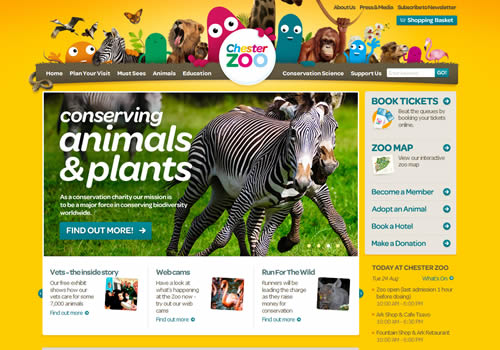A webpage for Chester Zoo is depicted, featuring a vibrant and informative design aimed at helping visitors plan their trip. The background of the site is predominantly yellow, accented by a touch of gray on the right side. At the top of the page, "Chester Zoo" is prominently displayed in a cheerful, multicolored font that grabs attention.

The main section of the webpage highlights various attractions and services offered by the zoo. Illustrated with pictures of zebras, the site offers a user-friendly experience with numerous options to become a member, adopt an animal, book a nearby hotel, or make a donation.

Links are clearly provided to help users navigate essential information such as downloadable maps, how to buy tickets, and other visitor services. The overall design is both engaging and functional, serving as a comprehensive guide for anyone looking to visit or support Chester Zoo.